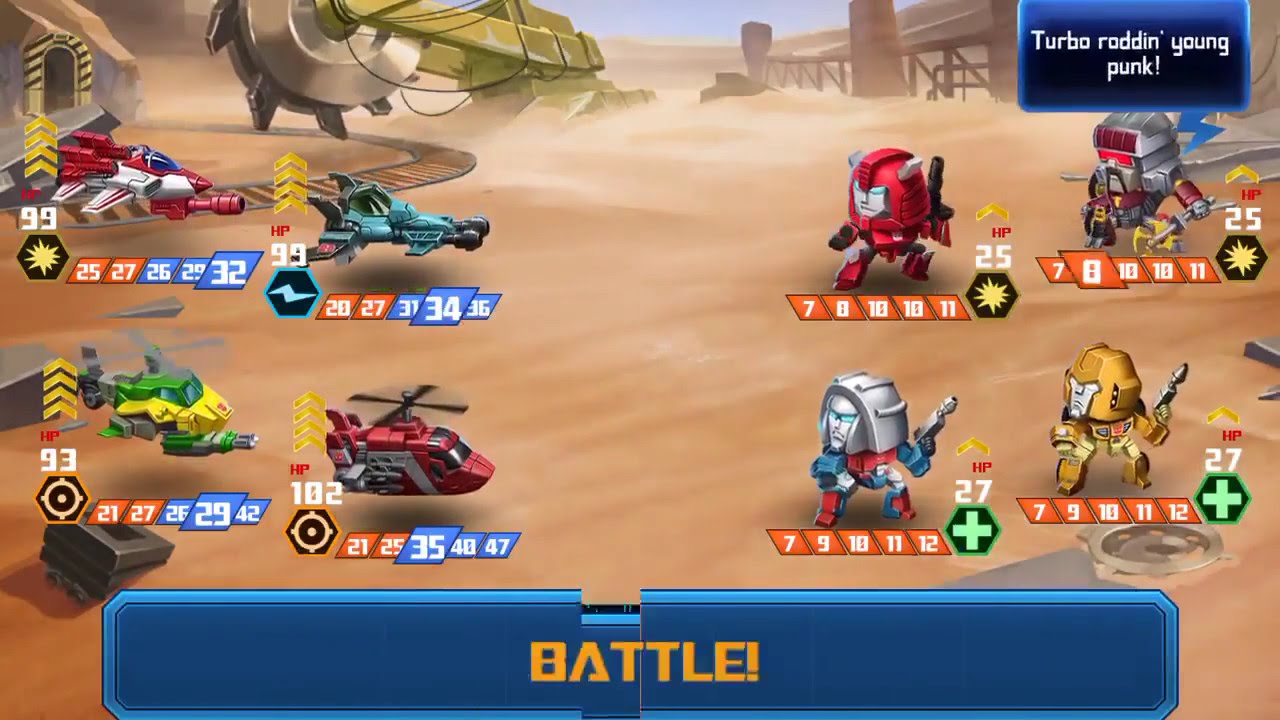This is an image from a video game that appears to be designed for younger players. The scene is set in a desert, characterized by sand dunes and an odd truck with a giant blade in the background. The main focus of the image is a 4v4 battle between two groups: four colorful vehicles on the left and four cartoon-like, robotic characters on the right.

On the left side, there are four differently colored vehicles—a red helicopter, a green and gray aircraft, a green and yellow craft, and a red and gray vehicle. Underneath each vehicle, there are orange and blue boxes with white numbers, which likely indicate stats or health points.

Facing them on the right are four armoured characters that resemble soldiers or robotic figures with exaggerated, big heads and small bodies. They come in red, silver, more silver, and green, with another person in gold. Each character has numbers and health meters above them, as well as individual boxes displaying their stats.

The backdrop of this battle scene is an orange desert landscape, adding a warm tone to the environment. At the bottom of the image is a prominent blue bar that spans the length of the screen, featuring the word "Battle!" in large, bold, yellow letters.

In the top right-hand corner, a small blue box contains white text listing names like Turbo, Radden, Young, and Punk, which could be character names or user handles. The image is rectangular, longer horizontally, resembling a typical mobile game screen.